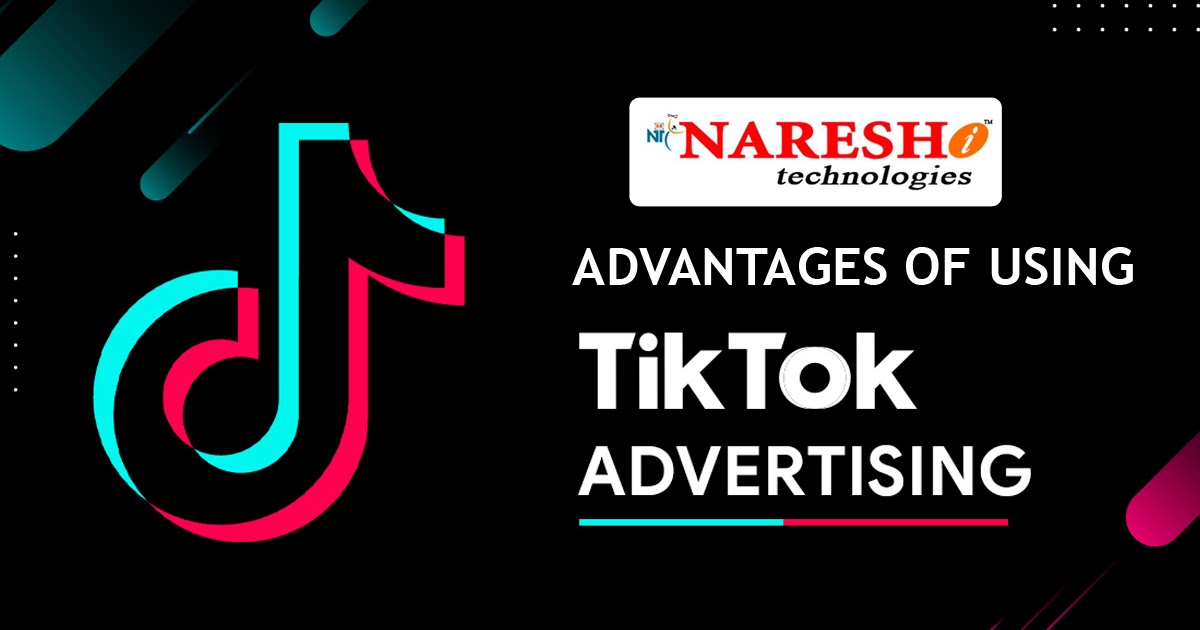### Detailed Caption

This image appears to be an advertisement banner, possibly sourced from a digital platform or flyer, given the design elements and layout. The predominant background color is black, providing a sharp contrast to the other elements, thus helping them stand out. 

On the left-hand side of the banner, there is a prominent, large TikTok icon, which is immediately recognizable and draws attention. Toward the middle-right of the banner, there is a white rectangle containing red text that reads, "Nourish Information Technologies." Directly below this, on the black background, white text states, "Advantages of Using." The next line continues with "TikTok" in white, and the subsequent line features the word "Advertising" in a visually striking manner. The word "Advertising" is underlined with TikTok's signature colors: teal and hot pink.

Additionally, the far left side of the banner showcases a vertical column of eight white dots, neatly aligned along the edge. Complementing this design, the upper right-hand corner features a horizontal row of 14 white dots, adding to the overall balance and aesthetic appeal of the banner.

The combination of these elements suggests a focus on highlighting the benefits of advertising on TikTok, leveraging the platform's branding colors and visually engaging design elements to capture interest.